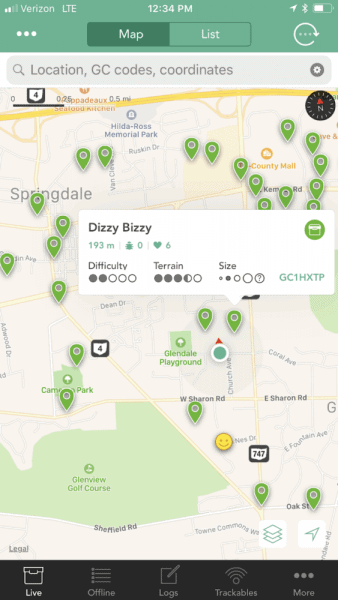Screenshot of a mobile application interface at 12:34 PM, with indicators showing it is connected to Verizon LTE and Bluetooth. The top right corner features a three-dot menu icon. Below that are tabs labeled "Map" and "List," along with a refresh button and a menu icon with three horizontal lines.

The center of the interface includes a search bar with options for location, GC codes, and coordinates. It also displays settings and search icons. The map in the background is populated with numerous green location markers. 

On the right side, there's a compass icon, two overlapping squares displaying the number "4" suggesting a route, and another square showing "747" with a smiley face icon. Additionally, the map details a location titled "Dizzy, Busy," noted as being 193 meters away. 

A heart with a “6” next to it and an icon of a person with a “0” follow, indicating search tags or metadata. The difficulty level is represented by two out of five circles, and terrain difficulty is marked by three and a half out of five circles, depicted with varying degrees of shading.